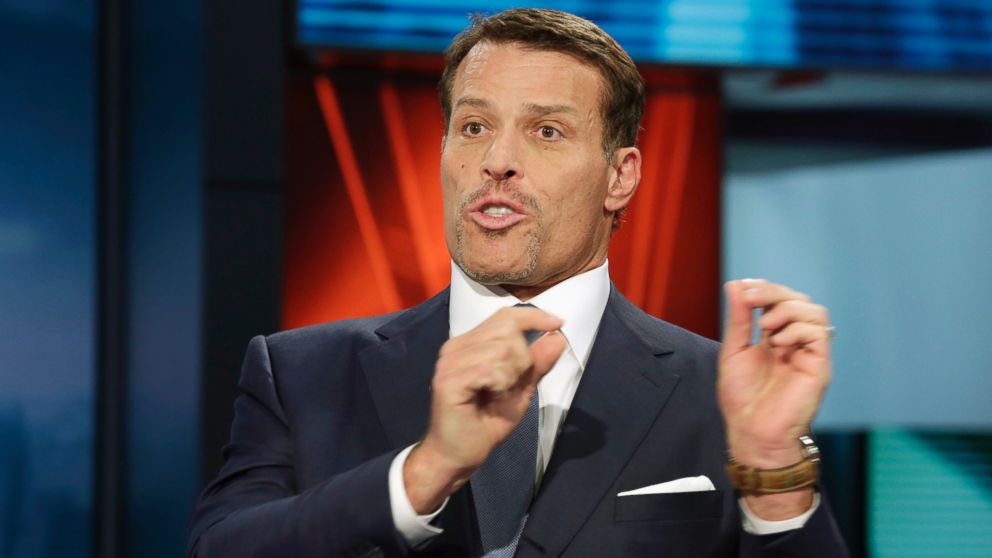This photograph features motivational speaker Tony Robbins, who appears to be in his 40s. He is captured mid-speech, with his arms raised and hands gesticulating, and his eyes wide open, looking slightly to the side with his mouth open. He is dressed impeccably in a dark blue suit with a white handkerchief neatly tucked into his breast pocket, a white collared shirt, and a light blue tie. Tony Robbins' short brown hair is combed to the side, and he sports a finely trimmed goatee that is more grey than brown. On his left wrist, he wears a silver wristwatch with a brown leather strap. The background is a colorful mix of red, green, blue, and orange hues, resembling a studio setup, likely for a talk show or a news program.